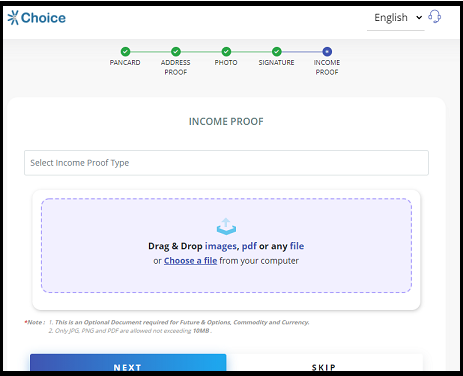The image is a detailed screenshot of a software interface, likely an online form. The interface is displayed in a landscape orientation with a black border that is thicker at the top and bottom. The background of the form is white.

In the top left corner, the word "Choice" is prominently featured in blue text, next to an icon resembling a partial circular shape with six blue lines radiating outward. Across the top right corner, there is a drop-down menu labeled "English" with an adjacent blue headphones icon. 

Below this header section, a horizontal progress bar is visually divided into sections. Each section is marked with a task title and its status, symbolized by green check marks and a blue circle. The tasks listed are: PAN Card, Address Proof, Photo, Signature, and Inca Proof. The current task is "Inca Proof," as indicated by the progress bar and text below it.

The section for "Inca Proof" is identified by its title in gray letters on a white background. Beneath this, there is an input field labeled "Select Inca Proof Type." Directly below the input field, a blue rectangle with rounded borders and a thin dashed blue line prompts users to "Drag and drop images, PDF or any file or choose a file from your computer." The phrase "Choose the file" is a clickable hyperlink accompanied by a blue icon depicting a box with an arrow pointing upwards.

At the very bottom of the page, there are two buttons: a blue button with white text reading "Next" on the left and a white button with black text reading "Skip" on the right.